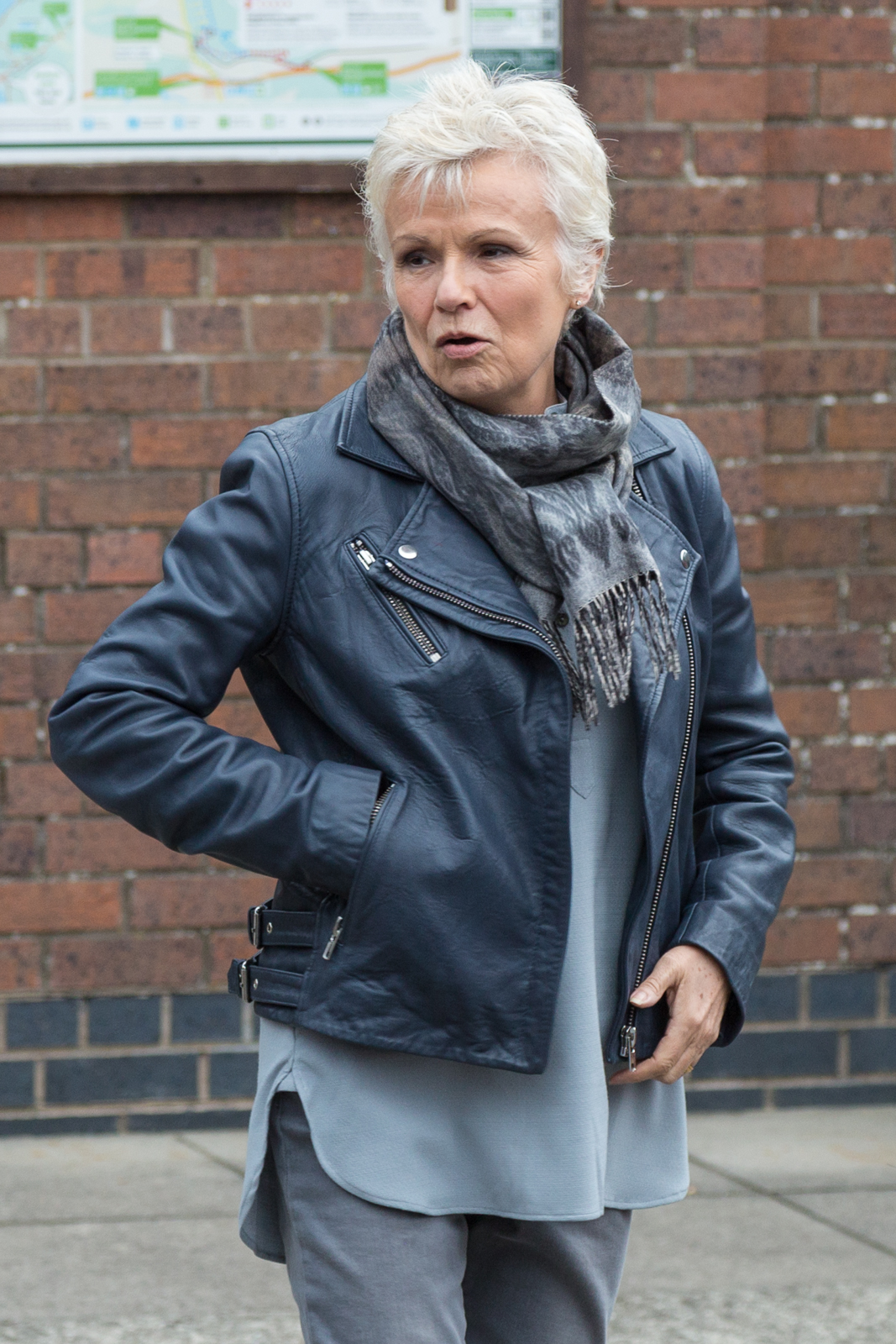The image features actress Julie Walters standing outdoors in front of a predominantly red brick wall with a gray brick foundation. A large concrete sidewalk, divided into several rectangular concrete panels, extends before her. Julie Walters, with short white hair, is looking to her right and is dressed in a dark blue leather jacket, which is unzipped to reveal a light blue, longer-length shirt. She also wears gray pants and a dark and light gray scarf, with her right hand tucked into the jacket pocket. In the background, partially obscured and blurry, is a framed map affixed to the wall, hinting at a location indicator.